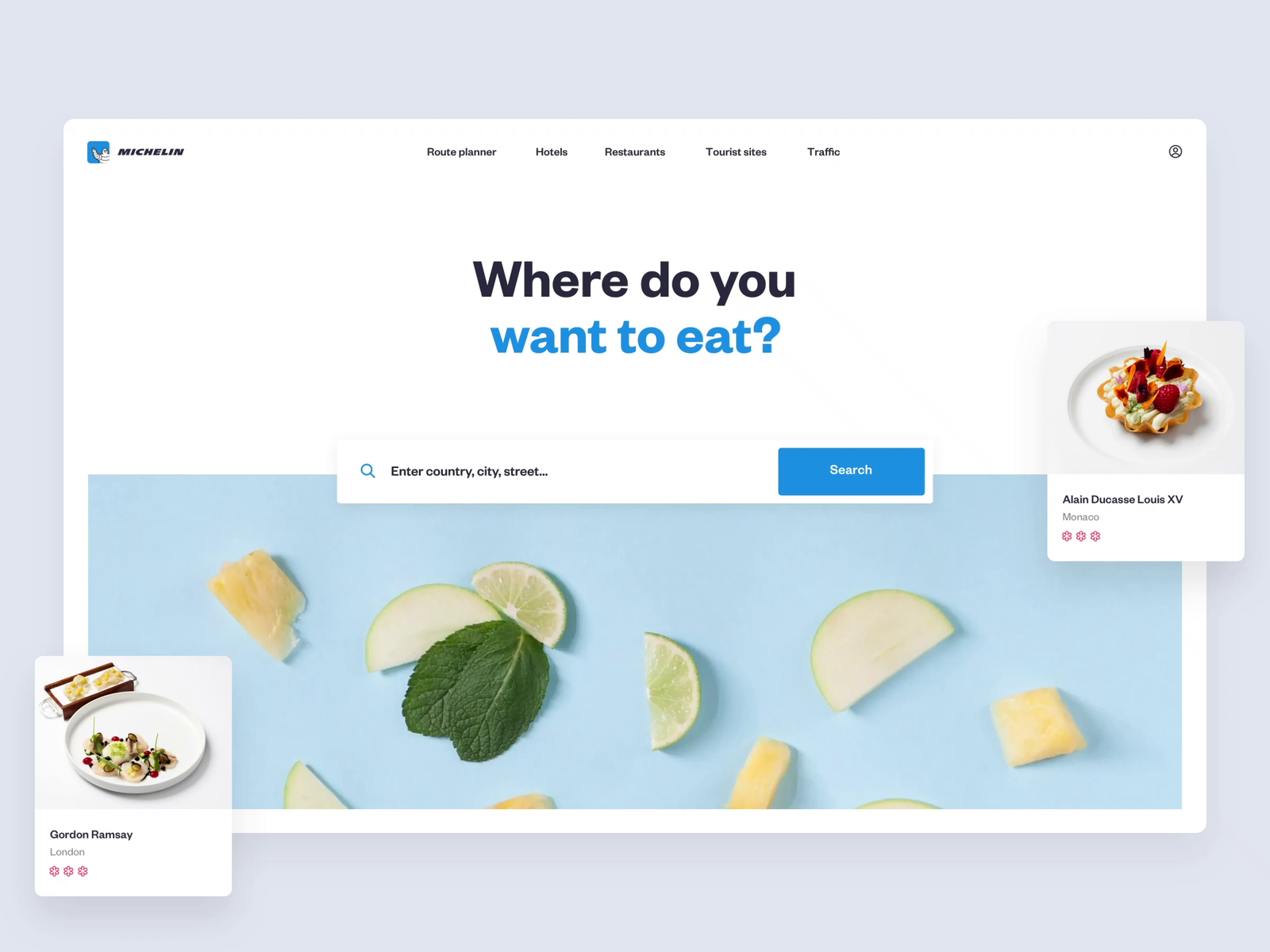The webpage displayed in the image is a Michelin website, identified by the "Michelin" logo in the top left corner of the main webpage. The logo features a white icon on a blue background. The website's outer border has a slightly grey hue, framing the central content area. At the top, black text labels several tabs: Route Plan, Hotels, Restaurants, Tourist Sites, and Traffic. In the top right corner, there is a profile icon.

Prominently in the middle is the text prompt, "Where do you want to eat?" displayed with "Where do you" in black text and "want to eat" in blue text. Below this, there is a search box with placeholder text that reads "Enter country, city, street," followed by a blue search button on the right-hand side.

On the right side of the main content area, there is an image of a dish associated with the text "Alain Ducasse, Louis XV, Monaco." The featured dish in the image consists of vibrant yellow, red, and white colors. Another food image appears on the bottom left of this section, labeled "Gordon Ramsay," indicating the famous chef.

At the bottom of the main webpage, the background transitions to a slightly light blue color, adorned with images of lemons, green leaves, and a lemon sliced into three segments.